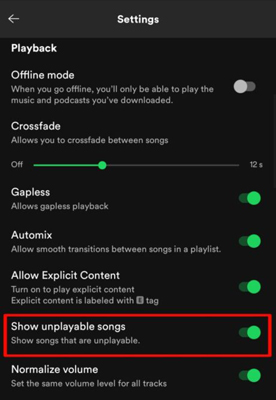This is a detailed description of the settings page on the Spotify mobile app, presented in dark mode with white text on a nearly black background. At the very top, the word "Settings" is displayed in white on a dark grey background, establishing the page's title.

The first category on this page is "Playback." The first option within this category is "Offline Mode," and the toggle next to it is set to off. The text description beneath this option explains, "When you go offline, you'll only be able to play the music and podcasts you've downloaded."

Next, there is an option for "Crossfade," which includes a slider allowing users to adjust the crossfade length between songs. The slider ranges from "Off" on the left to "12 seconds" on the right. In this instance, the slider is set to approximately one-third of the full length, indicating a crossfade duration of about 4 seconds.

Following Crossfade, the next category is "Gapless Playback," which enables uninterrupted playback between songs. The toggle for this option is green, indicating it is turned on.

The "Auto-mix" option follows, allowing smooth transitions between songs in a playlist. This toggle is also green, indicating that this feature is enabled.

Next is the "Allow Explicit Content" option, which, when turned on, permits the playback of explicit content labeled with an "E" tag. This toggle is green, showing that it is active.

Then there is the "Show Unplayable Songs" feature, which displays songs that are unplayable. This toggle is also green, signifying it is turned on, and there is a red rectangle surrounding it to draw attention.

The final option on this screen is "Normalize Volume," which equalizes the volume level for all tracks. This toggle, like the others, is set to green, indicating that the feature is activated.